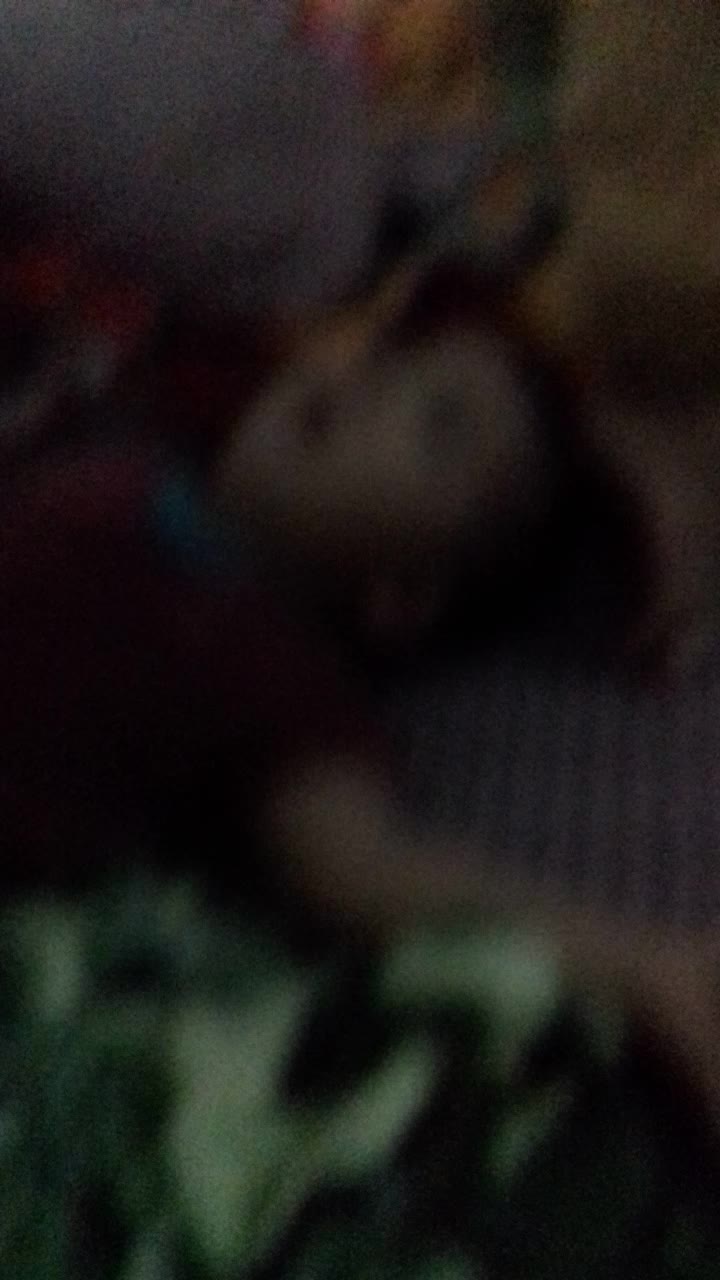The image portrays a grainy, dimly-lit scene filled with dark and blurry shapes, creating an unsettling and gritty atmosphere. At the lower part of the picture, there is a crumpled green object, possibly a piece of cloth or a comforter, with a slightly darker green hue on the left side. Above this, a brown tube-like shape can be discerned. The middle of the image features a blue and gray striped element, possibly bedding, upon which lies a child looking up toward the top left corner, though not directly at the viewer. The child's face is pale, partially visible amidst the blurriness, with faintly discernible hair blending into the murky background. The child appears to be wearing a short-sleeved, purplish shirt, and extending towards the right is what seems to be her pale arm. In the upper right portion, a brown round shape is visible, while the upper section of the image is divided between gray on the left and brown on the right, adding to the indistinct and mysterious quality of the photograph.